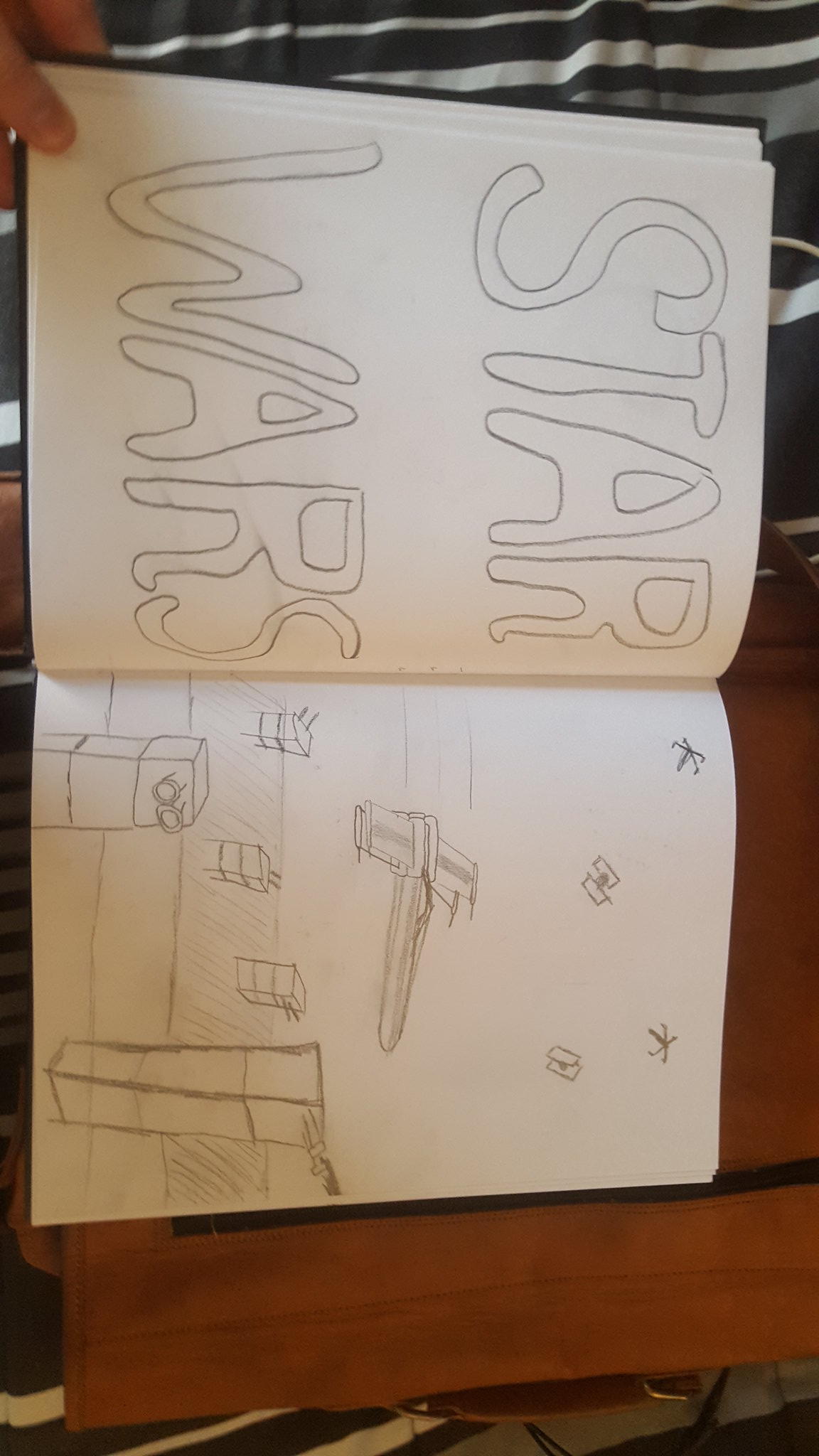This photograph captures a detailed sketchbook laid open on a wooden desk, with someone holding it in place by the corner using their thumb. The sketchbook is viewed at an angle, adding an interesting dynamic to the image. On the upper left side of the open pages, "Star Wars" is prominently written in large bubble letters, meticulously sketched in pencil across the whole page. The opposite page, oriented towards the bottom right, features an intricate pencil drawing depicting a space battle. A starship, likely the iconic X-wing fighter used by Luke Skywalker, soars through the scene with dynamic lines emphasizing its motion. Background details include enemy fighters and astronomical elements like stars, evoking the desperate battle against the Death Star. The entire scene is set against the simple backdrop of a wooden surface under dim lighting, adding a rustic touch to the photograph.